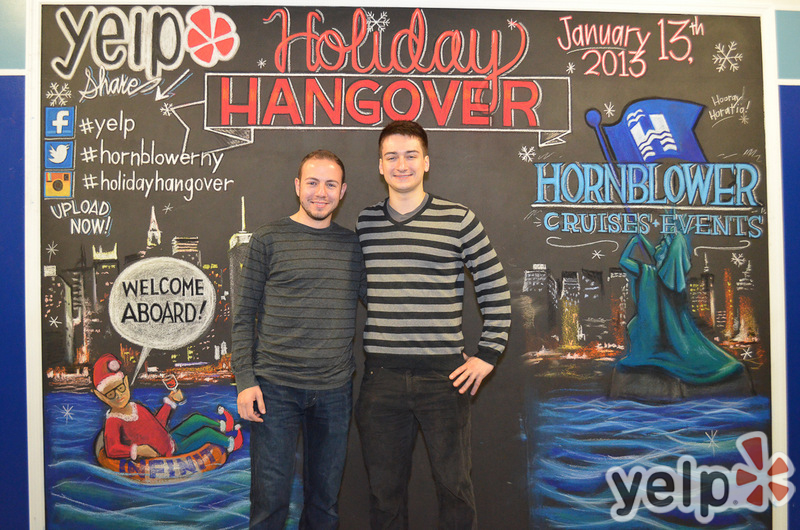The image captures two men standing side-by-side, posing in front of a decorative signboard adorned with various logos and a detailed illustration. The signboard prominently features the words "Holiday Hangover" at its center and includes multiple social media references such as Yelp, Facebook, and Twitter with hashtags like #HornblowerNY and #HolidayHangover. Both men are wearing long-sleeve shirts with horizontal stripes; the man on the left sports a charcoal gray shirt with thin black stripes and blue jeans, while the man on the right is in a light gray sweater with thick black stripes and black jeans. Both men have short hair and are smiling at the camera.

The backdrop behind them, which sets the festive theme, displays a colorful oceanfront cityscape. This includes a humorous illustration of Santa in a red and green outfit floating in an inner tube on what appears to be a river, sipping a drink, with a speech bubble that reads "Welcome aboard." Additionally, the backdrop has a city skyline and what resembles the Statue of Liberty, uniquely depicted as blowing a horn. Text elements on the backdrop also highlight "Hornblower Cruises Events" on the right side with a blue sign, and the date "January 13, 2013" in pink at the top.